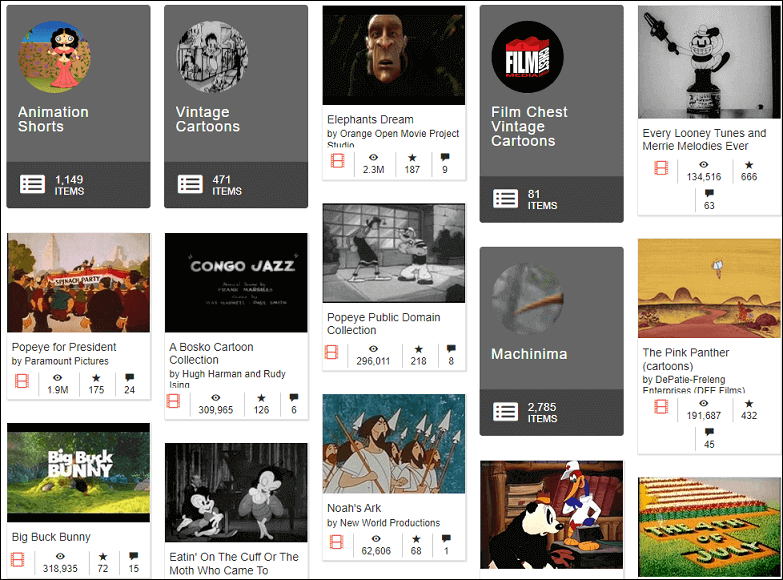**Image Description: Screenshot of a Video Collection Interface**

The screenshot showcases a video collection interface categorized into various sections. Prominently featured is "Elephant's Dream" by Orange Open Movie Project Studio, highlighted by an eyeball icon indicating it has amassed 23 million views, a star icon denoting 187 likes, and a comment icon representing no comments.

Adjacent to it, there is a segment titled "Animation Shorts" containing 1,149 items, and "Vintage Cartoons" with 471 items. A noteworthy mention under the "Vintage Cartoons" section is "Pawpaw for President" by Paramount Pictures, which has garnered 1.9 million views, 175 likes, and 24 comments.

The collection also includes "Every Lonely Looney Tunes and Merry Melodies Ever," which has accumulated 134,516 views, 666 likes, and 63 comments.

Additionally, there's the "Bosco Cartoon Collection" by Hugh Harman and Rudy Ising, which has collected 309,965 views, 126 likes, and 6 comments.

The interface further highlights categories such as "Film," "Chess," and a subset of "Vintage Cartoons" with 81 items. Each section is represented with distinct visuals and numerical indicators outlining the viewer engagement through icons for views, likes, and comments.